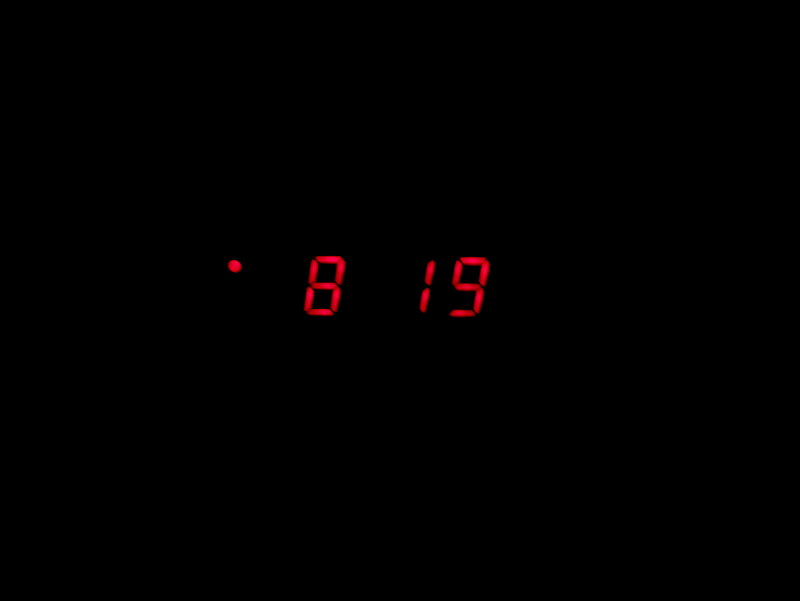In the image, everything is shrouded in near-total darkness, creating a sense of eerie obscurity. The only visible detail is a set of glowing red digital numbers "8" and "19" alongside a single red dot. These elements suggest that we are looking at the display of an old-fashioned digital alarm clock, likely in a completely darkened room. The lack of any other visible details or surrounding context makes the numbers and dot appear as if they are floating in mid-air, adding to the unsettling atmosphere of the scene. The dot might indicate that the alarm is set or denote the AM/PM setting, but without more context, it's impossible to determine its exact function. The image taps into a stark and minimalist aesthetic, defined solely by the faint red illumination against a pitch-black background.